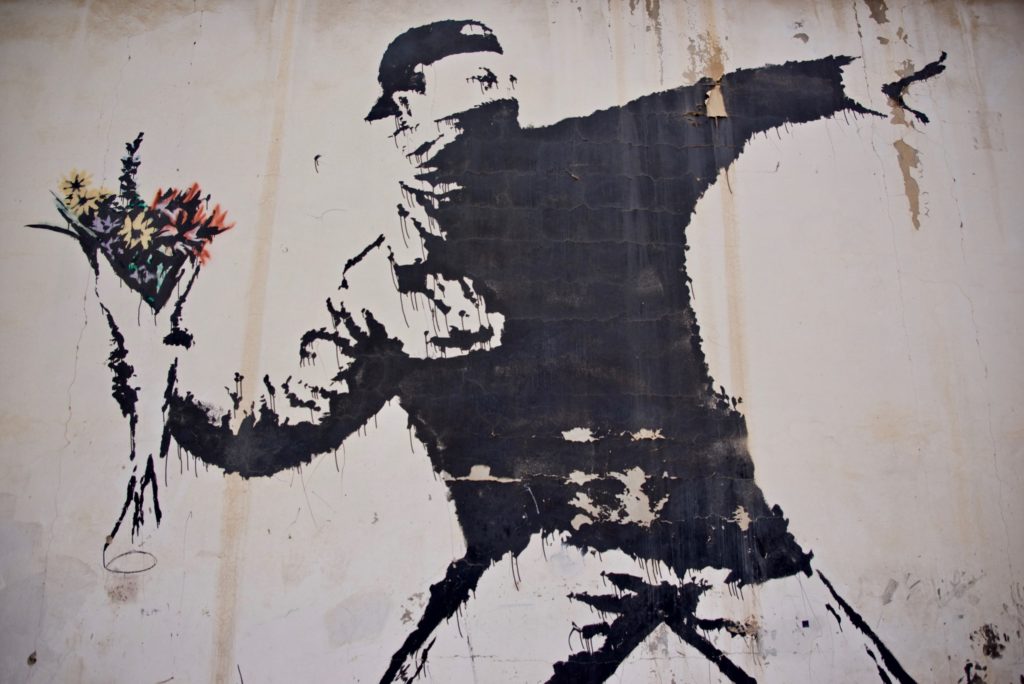A striking black and white graffiti-like artwork appears on a dilapidated, spalling wall, where the white paint is peeling off, revealing the rough texture underneath. At the center of this detailed mural, a man is depicted in a dramatic pose. He wears a black baseball cap turned backward, a long-sleeved black shirt, and white pants. His face is partially obscured by a dark bandana or scarf covering his nose and mouth, leaving only his intense eyes visible, which convey a sense of anger. The man's left hand is raised pointing outward, while his right hand, pulled back as if about to throw something, holds a bouquet of vividly colored flowers—the only splash of color in the otherwise monochromatic image. The bouquet includes yellow, purple, and red flowers, resembling Asteraceae and black-eyed Susans. The artwork, vividly realistic and brimming with emotional tension, ironically replaces what might be a weapon with flowers, juxtaposing the aggressive stance with the gentleness of the floral arrangement. The brick wall beneath the peeling paint adds a raw, urban texture to the impressive street art.